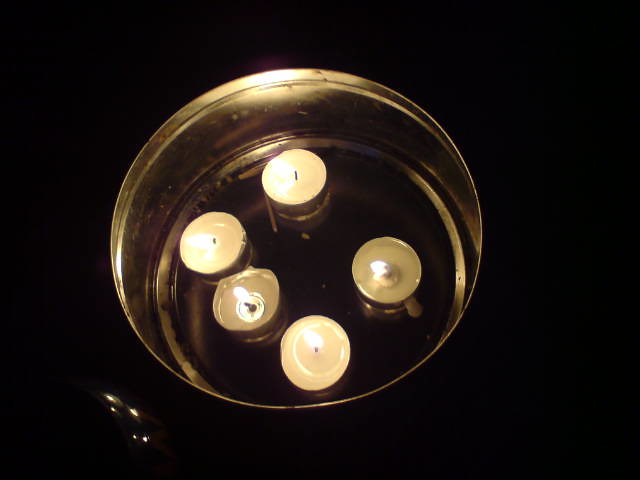The image depicts five lit tea light candles situated inside a large steel pail or chafing dish. Each small candle is encased in its own individual metal holder. Two of the candles are almost completely melted, their wax turned liquid, while the other three have varying degrees of unburned white wax remaining. All the candles produce a white flame. The interior of the steel container shows wax accumulating at the bottom. The background is predominantly black, providing stark contrast, with the lower left corner marked by a reflection appearing as a few small, shining white dots—possibly from the handle of the steel dish.